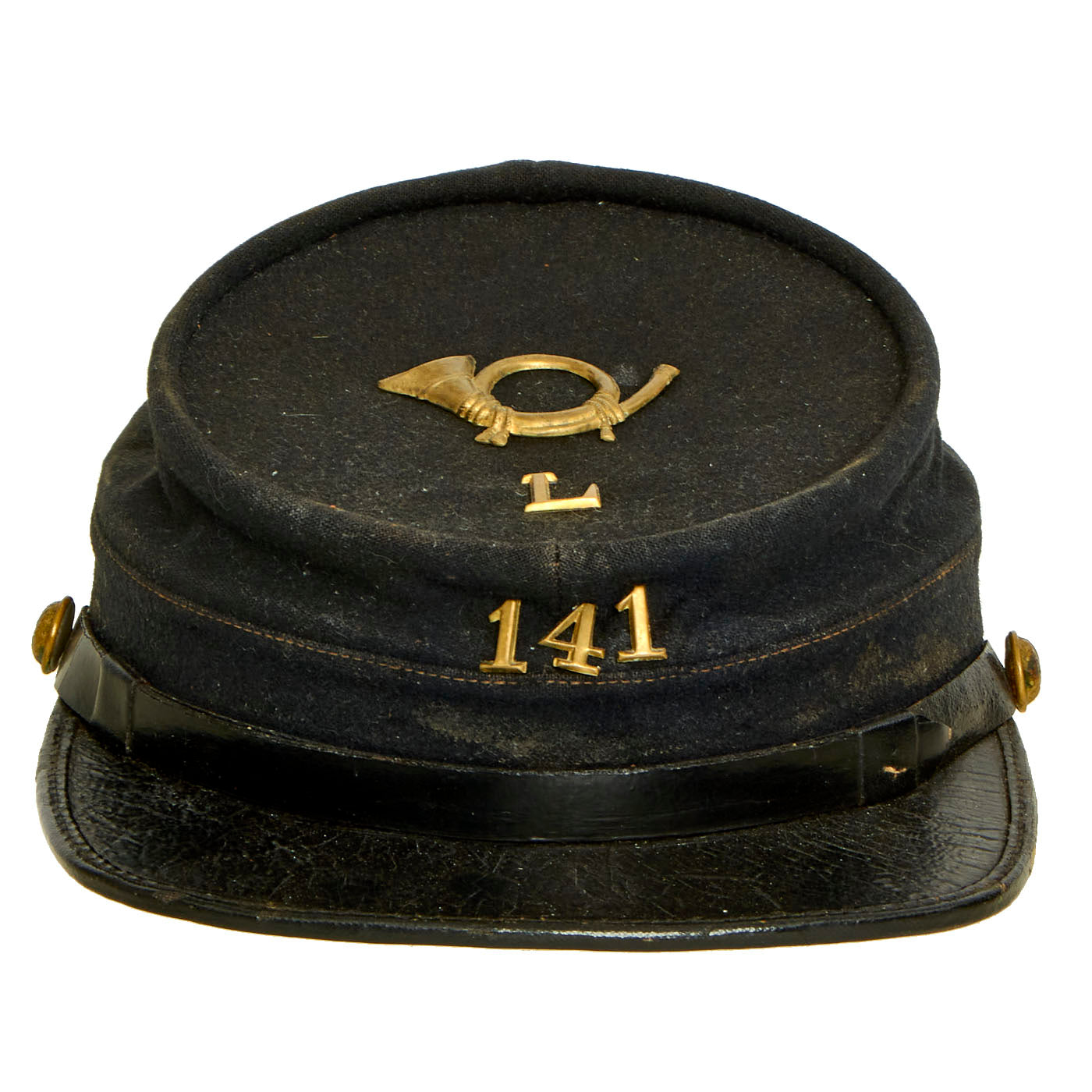This is a detailed stock photograph of an antique, dark military hat that prominently features several gold accents. The hat, which may be black or a very dark green, has a somewhat smushed appearance. It has a rounded top with a flat edge and an overhanging brim. Just above the brim, a black leather or fabric band encircles the hat, adorned with decorative gold buttons on either side near the temple area. The hat also displays significant brass elements: a gold letter "L" and a gold pin depicting a French horn, with the mouthpiece on the right and the bell on the left. Below these decorations, the numbers "141" are depicted in gold. The hat's design suggests it could be part of a military or orchestral uniform, given its structured style and ornamental gold elements.